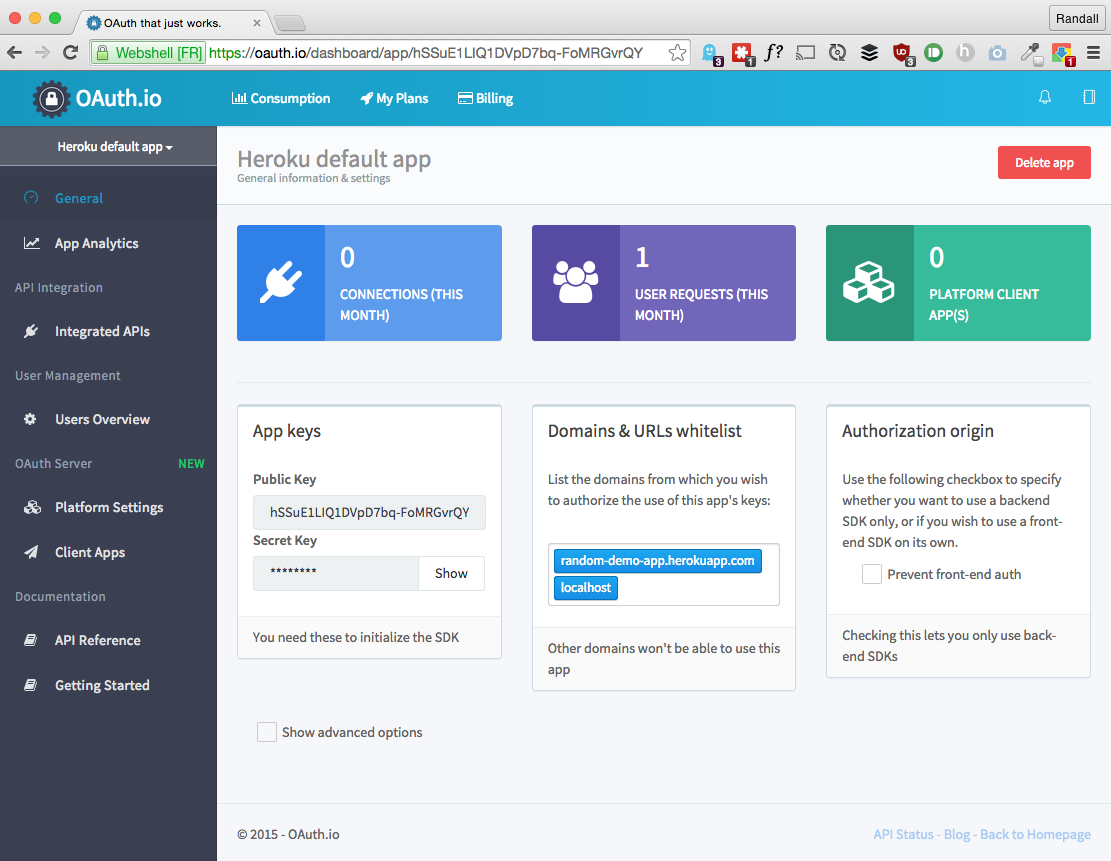The image showcases a computer screen, likely from a developer's dashboard, displaying an OAuth management interface. At the very top of the screen, familiar red, yellow, and green buttons are visible, commonly found on browser windows for closing, minimizing, and maximizing.

Below these, a browser tab titled "OAuth that just works" is open. The interface underneath begins with a search bar labeled "web show," alongside an "FR" marker and a website URL. Directly below, the heading "OAuth.io" is featured prominently, followed by navigation tabs labeled "DD consumption," "my plans," and "billing."

The main content area displays detailed app information:
- **App Name**: Heroku Default App
- **Action**: A red "Delete App" button is available.
- **Usage Statistics**: 
  - 0 connections this month
  - 1 user request this month
  - 0 platform client apps

Further down, a section titled "App Keys" reveals the technical credentials required for initializing Secure OAuth Kit (SOK):
- A public key is provided in full.
- A secret key is obscured by a series of asterisks, with an option to click "show" to reveal it.

Additional configurations include:
- **Domain and URL Whitelist**: Instructions for listing domains authorized to use the app's keys. Currently listed are:
  - random-demo-app.herokuapp.com
  - localhost

Towards the end, there is a section labeled "Authorization Origin" that finalizes the displayed information.